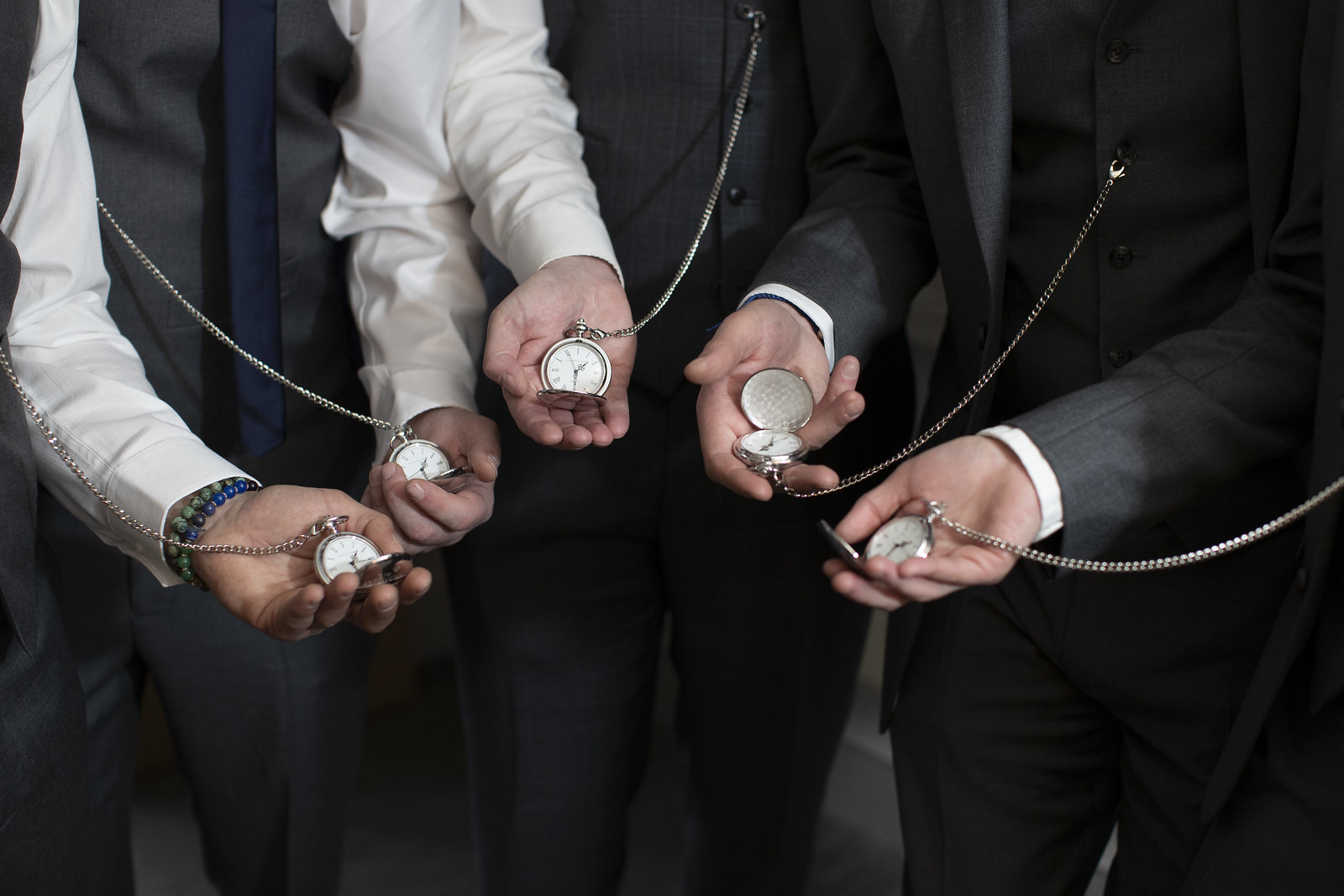In this detailed image, we see five men, gathered in a semicircle, all dressed in formal attire, possibly for a wedding. Their outstretched hands prominently display identical open pocket watches, each attached to their suits via a chain. The men are primarily dressed in black suits or black shirts, with white undershirts visible for some of them. Specific details among the attire include one man on the left wearing a light black shirt with a blue tie that extends past his shirt, and another on the far left who wears bead-like wrist accessories colored blue and green. The middle right individual dons a black jacket with white cuffs and black pants, while the central figure sports a black shirt and black pants without a jacket. The coordinated display of pocket watches, all uniformly styled and open to show the time, suggests a ceremonial or commemorative occasion, reinforcing the impression that this image captures a special moment, likely among a groom and his groomsmen.